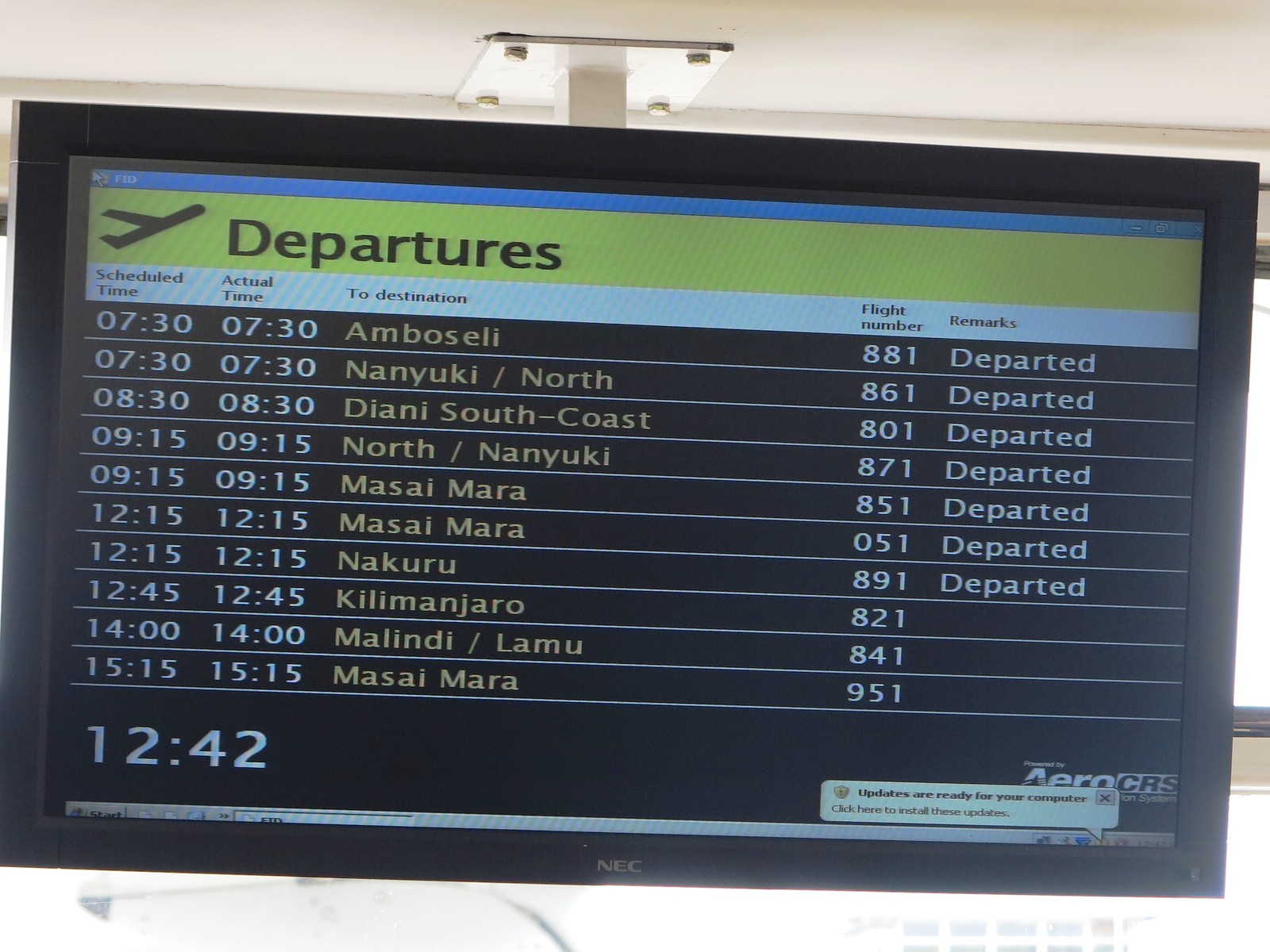The image depicts a rectangular, horizontally aligned departure board from an airport. The board is framed with a black border like a television screen and features a distinctive green stripe along the top with the word "Departures" in black, accompanied by an airplane icon. Directly beneath this banner, the board is organized into several columns displaying crucial departure information: "Scheduled Time," "Actual Time," "To Destination," "Flight Number," and "Remarks." 

The display lists multiple destinations with detailed schedules starting from 7:30 AM to 3:15 PM (written as 1515). Notable locations listed include Amboseli (Flight 881, departed at 7:30), Newquay North (Flight 861, departed at 7:30), Diane South Coast (Flight 801, departed at 8:30), North Newquay (Flight 871, departed at 9:15), Masai Mara (Flight 851, departed at 9:15), and another Masai Mara flight (Flight 051, departed at 12:15). Notably, flights to Kilimanjaro (Flight 821), Malindi Lamu (Flight 8401), and Masai Mara again (Flight 951) have yet to depart. The bottom left of the board prominently displays the current time as 12:42. Additionally, a pop-up box in the lower right corner indicates that updates are ready for installation on a computer. The image captures bolts from the supporting wall at the top and a segment of the white ceiling. Seven flights have departed, with three pending departures.